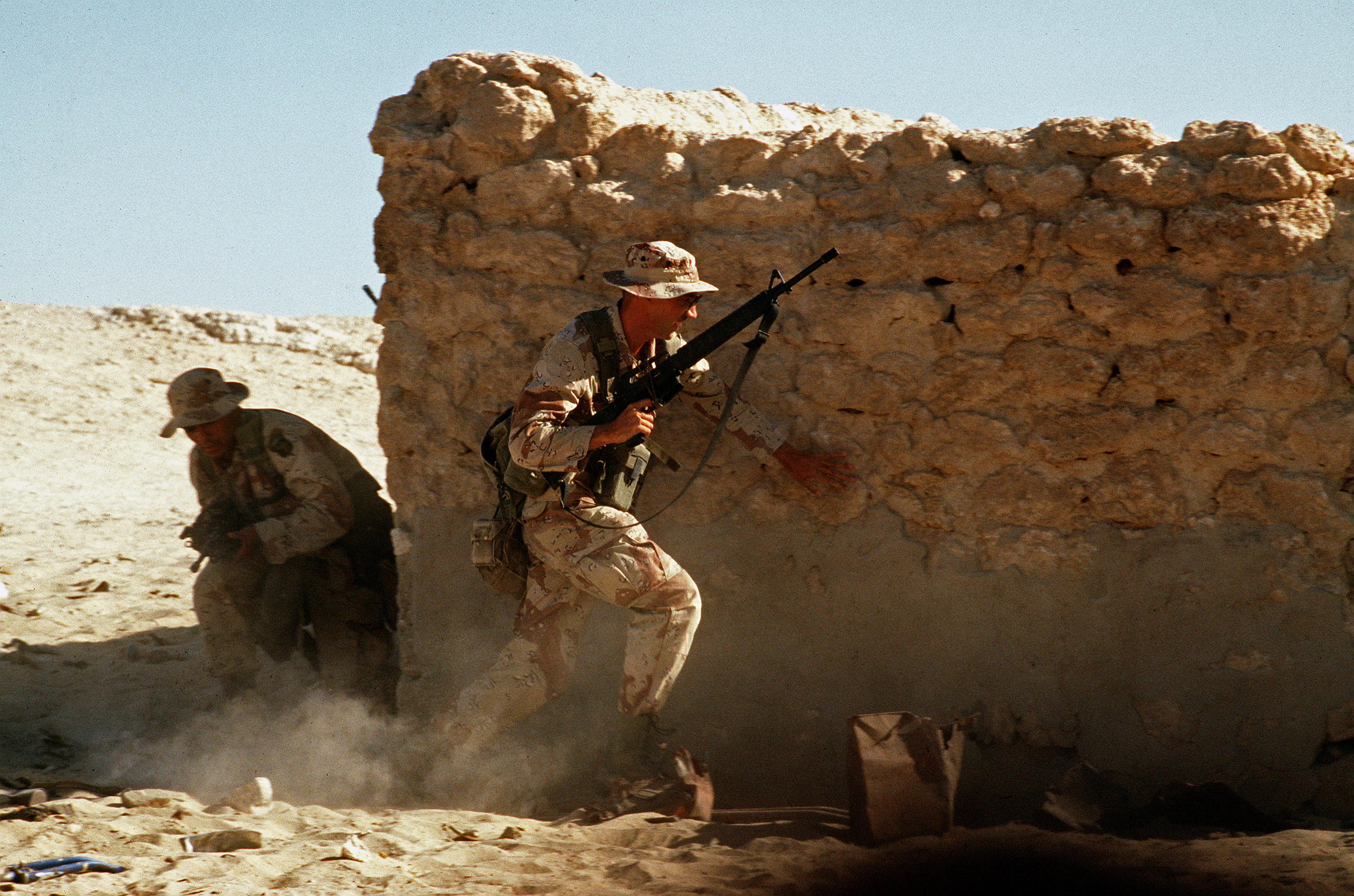A dynamic photograph captures two soldiers in the desert, navigating a war-torn landscape under a bright, sunny sky. In the foreground, the terrain is dominated by sand dunes and a tall, rustic stone wall that appears to be hand-built from stones and concrete. Shrouds of wind-swept sand create a smoky haze, adding to the scene's intense atmosphere. Both soldiers, dressed in light brown and tan desert camouflage uniforms and wide-brimmed bucket hats designed for sun protection, are armed with assault rifles. The soldier in the foreground, mid-run with his hand on the wall, carries a canteen and additional gear, and looks straight ahead with determination. A small bag lies at the base of the wall near him. The second soldier, partially obscured by the wall's corner, is also equipped with a rifle and mirrors the first soldier's cautious but urgent movement, looking down as he navigates the sandy terrain.